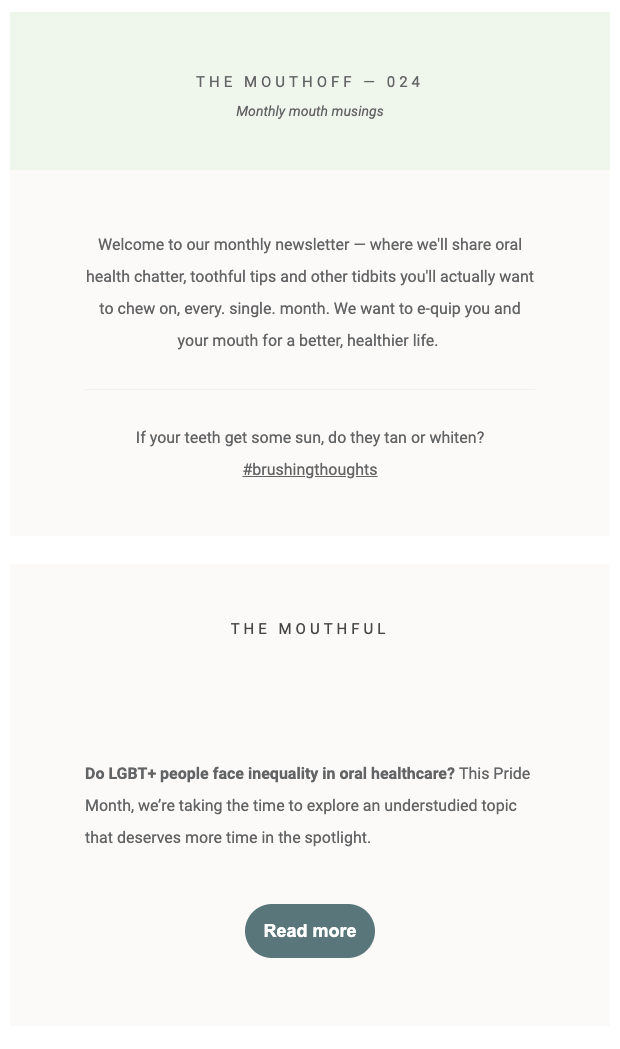**Detailed Descriptive Caption for Image:**

This image is a screenshot of a newsletter from a website called "The Mouthful." The screenshot features an edition titled "The Mouth Off 024," prominently displayed at the top in all caps, set within a light green box. Just below this title, in italicized text, it reads "Monthly Mouth Musings." 

Continuing downward, there is a white box containing the introductory message for the newsletter. It states: "Welcome to our monthly newsletter where we'll share oral health chatter, truthful tips, and other tidbits you'll actually want to chew on every single month. We want to equip you and your mouth for a better, healthier life." Notably, the phrase "Every single month" ends with a period after each word, and "equip" is written as "e-quip."

Following this section, a light green line separates the content, leading to a statement in dark gray font: "If your teeth get some sun, do they tan or whiten? #brushing thoughts," with the hashtag phrase underlined.

Lower on the page, there is additional content in another off-white box. At its top, "The Mouthful" is displayed again, followed by the question: "Do LGBT+ people face inequality in oral health care? This Pride Month, we're taking the time to explore an understudied topic that deserves more time in the spotlight." Below this text is a gray button with "Read More" inscribed in white font.

The overall design features a white background with off-white boxes and dark gray text, showcasing sections highlighted by light green accents. The structure and coloration provide clarity and emphasis on the newsletter's key topics related to dental health and LGBTQ+ issues within the context of oral healthcare.